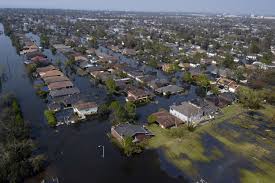This color photograph, taken from a drone in landscape orientation, vividly depicts a residential area heavily submerged in water following a flood, likely after Hurricane Katrina. The aerial view showcases numerous rows and columns of houses inundated by dark floodwaters that reach halfway up the structures. The rooftops, appearing in varying perspectives from wide at the bottom right to narrow at the top left, hint at the extensive scale of the flooding, covering almost a hundred houses. Interspersed among the houses are tall green trees whose tops stick out from the water, along with patches of dark green moss floating on the surface. The streets between the houses have transformed into canals, their original forms obscured by the flood. The scene extends to a horizon of flat land with distant buildings under a grayish-blue, somewhat obscured sky. Overall, the composition provides a realistic and representational snapshot of the catastrophic impact of the flood on this community.